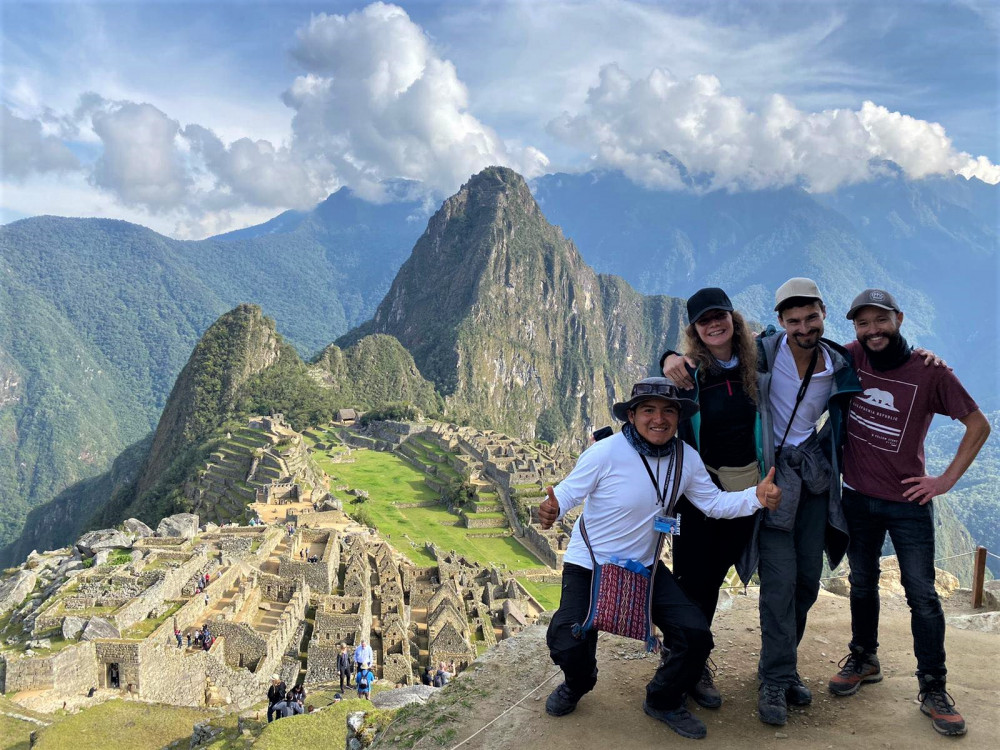The image depicts a vibrant group photo taken at the ancient ruins of Machu Picchu in Peru. Four individuals—three travelers and their guide—stand on the edge of a cliff, framed by the majestic backdrop of a sprawling, green mountain range that stretches into the clouds under a sky speckled with blue and gray hues. The ancient Incan architecture with its moss-covered stones and historical ambience is visible in the background, populated by other tourists also capturing their memories.

The group stands close together with arms around each other, beaming at the camera. The female, wearing a ball cap, black shirt, black pants, and a fanny pack, is flanked by three males. One man sports a red t-shirt, a beard, and a ball cap; another is dressed in a white t-shirt and ball cap with facial hair; and the guide, distinguishable by his white long-sleeve t-shirt, bucket hat, sunglasses, and a native-looking bag, smiles beside them. He also has a scarf and boots paired with black cargo pants. The final male in the group also wears a white long-sleeve t-shirt, along with a ball cap. The travelers, comfortably equipped for adventure in their hats, jeans, and boots, capture a moment of joyous camaraderie at one of the world's most renowned archaeological sites.